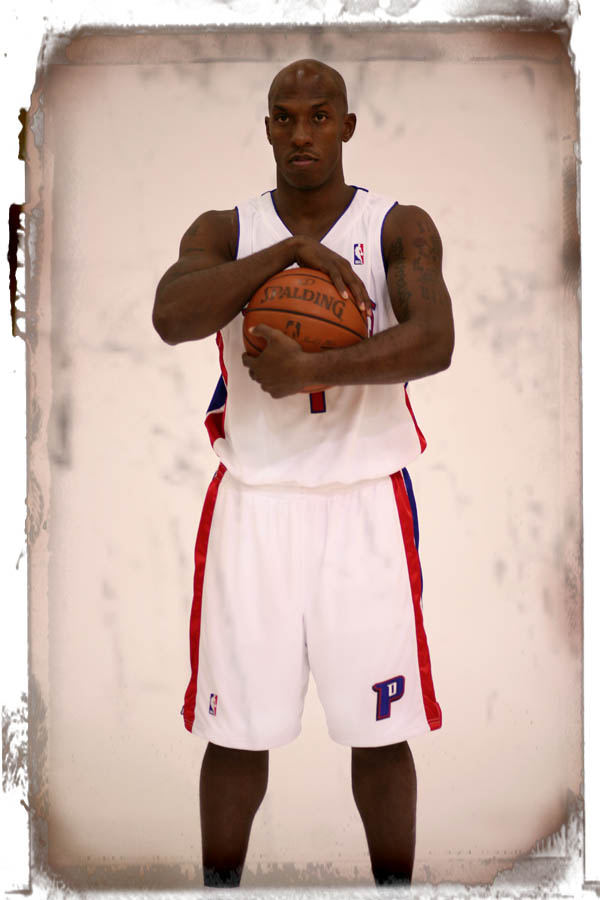This detailed color photograph features a young African American basketball player in his 20s or possibly early 30s, who appears to be an NBA athlete. The man is well-toned with a plethora of tattoos on his arms, and sports a bald or shaved head with a clean-shaven face. He is wearing a white basketball uniform consistent with the Detroit Pistons team colors: red, white, and blue. The uniform includes a white tank top and shorts, both adorned with red and blue accents. The number on the front of his tank top is mostly covered by the Spalding basketball he holds tightly in both hands, positioned in front of his chest. A blue 'P' is visible on the lower left side of his shorts, accompanied by red stripes on the sides. Additionally, a small, tricolored NBA logo is situated near his right knee. He stands composed and poised against a stark white, slightly grimy background that adds a dramatic contrast to the photo. The overall impression is of a well-built athlete, ready to take to the court for the Detroit Pistons.